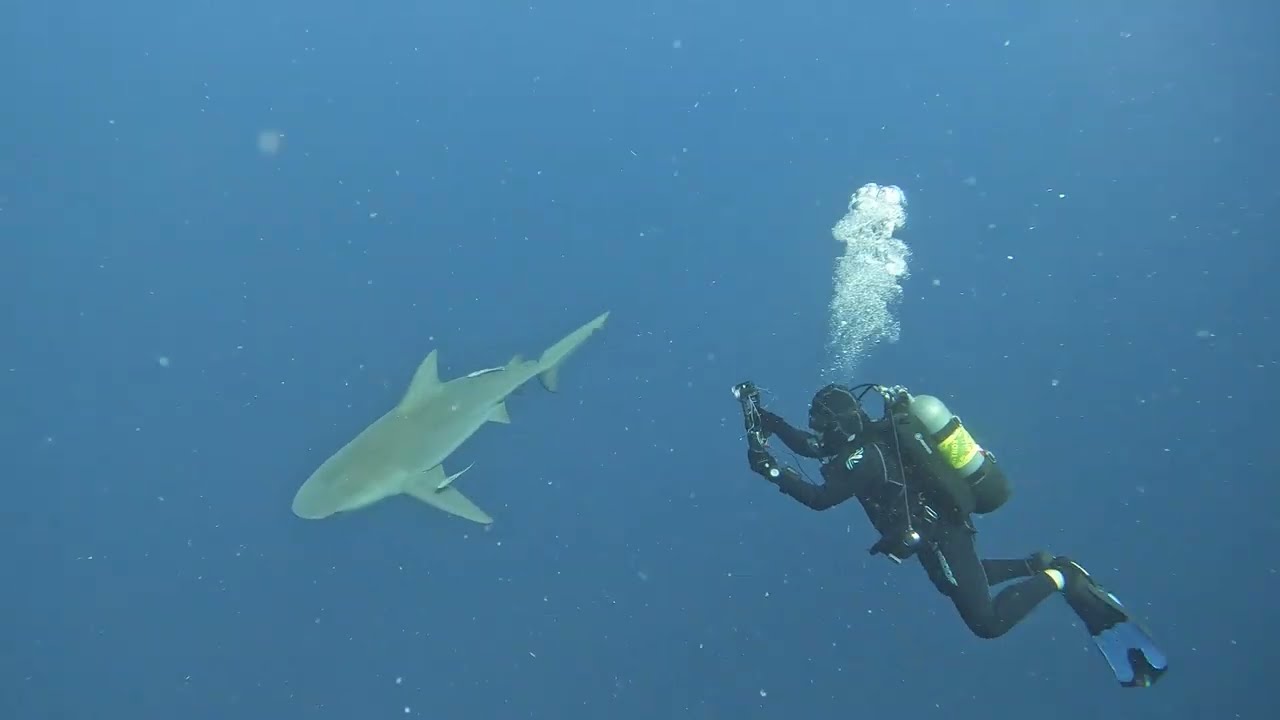In this detailed underwater scene, a scuba diver in a black suit with blue and black flippers explores the depths of a dark teal-colored ocean. Positioned to the slight right and bottom center of the frame, the diver is equipped with a steel air tank on their back and a large cloud of white bubbles streaming upwards from their air hose. They are holding a camera apparatus, aiming it towards a medium-sized gray shark that swims to their left, slightly further in the distance. The entire frame is immersed in the expansive field of medium blue water, devoid of visible boundaries, capturing the realism and vastness of the underwater environment.